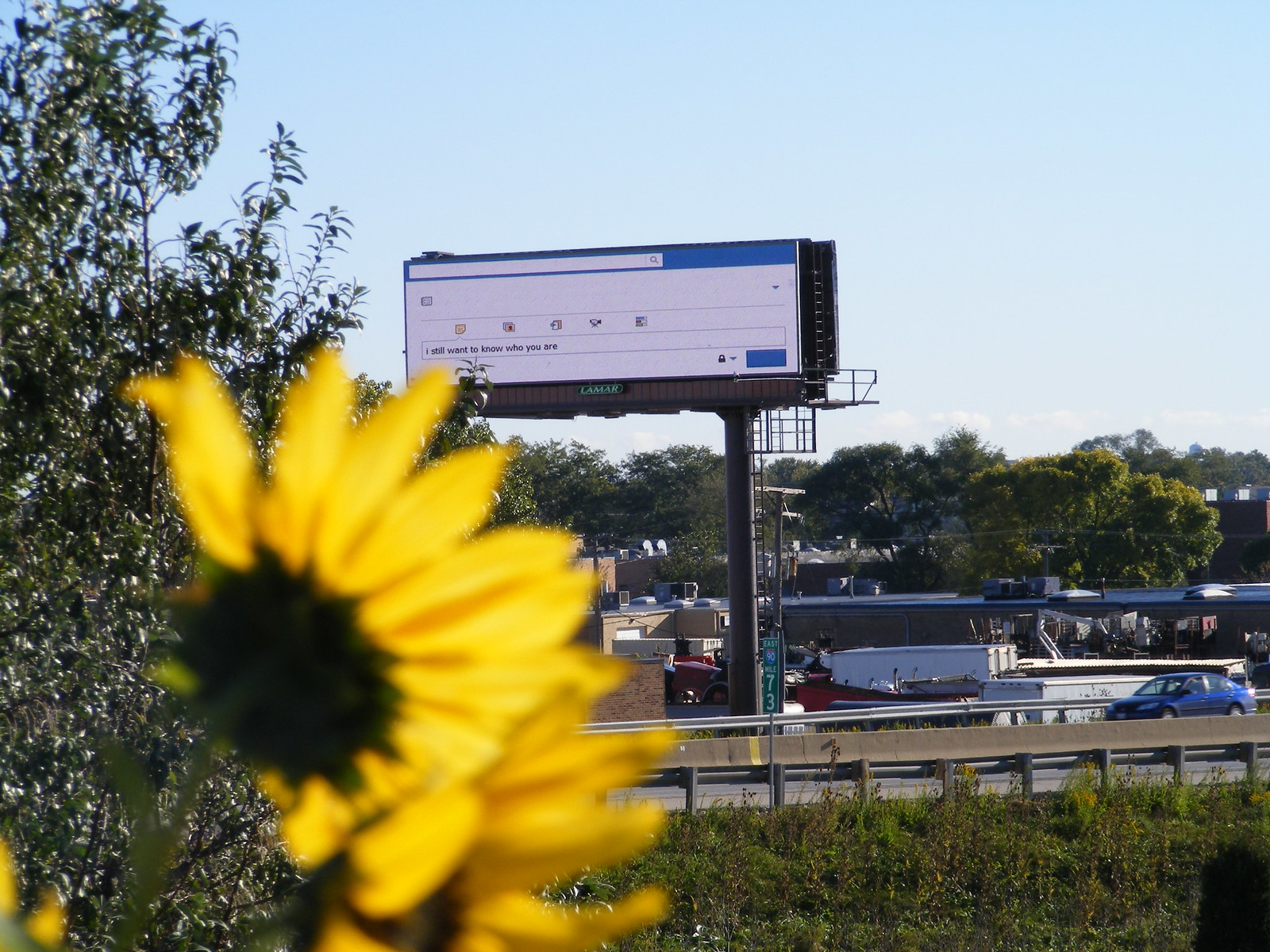A vibrant scene captured from a stationary viewpoint reveals a mixture of natural and urban elements along an interstate. In the lower left corner, detailed close-ups of yellow flowers show their delicate petals radiating from their stems. A large tree, accompanied by dense bushes, dominates the right side of the image, framing the scene subtly.

Beyond the foliage, a segment of the interstate curves off to the right, guiding the eye towards further urban features. A digital billboard, seemingly malfunctioning, displays a default page instead of an advertisement, hinting at a technological glitch. A blue car travels down the road, adding a hint of motion to the otherwise still scene.

In the distance, the tops of buildings and containers from trucks leave an industrial mark on the landscape. The horizon is softened by a backdrop of trees, merging the bustling infrastructure with nature's tranquility.